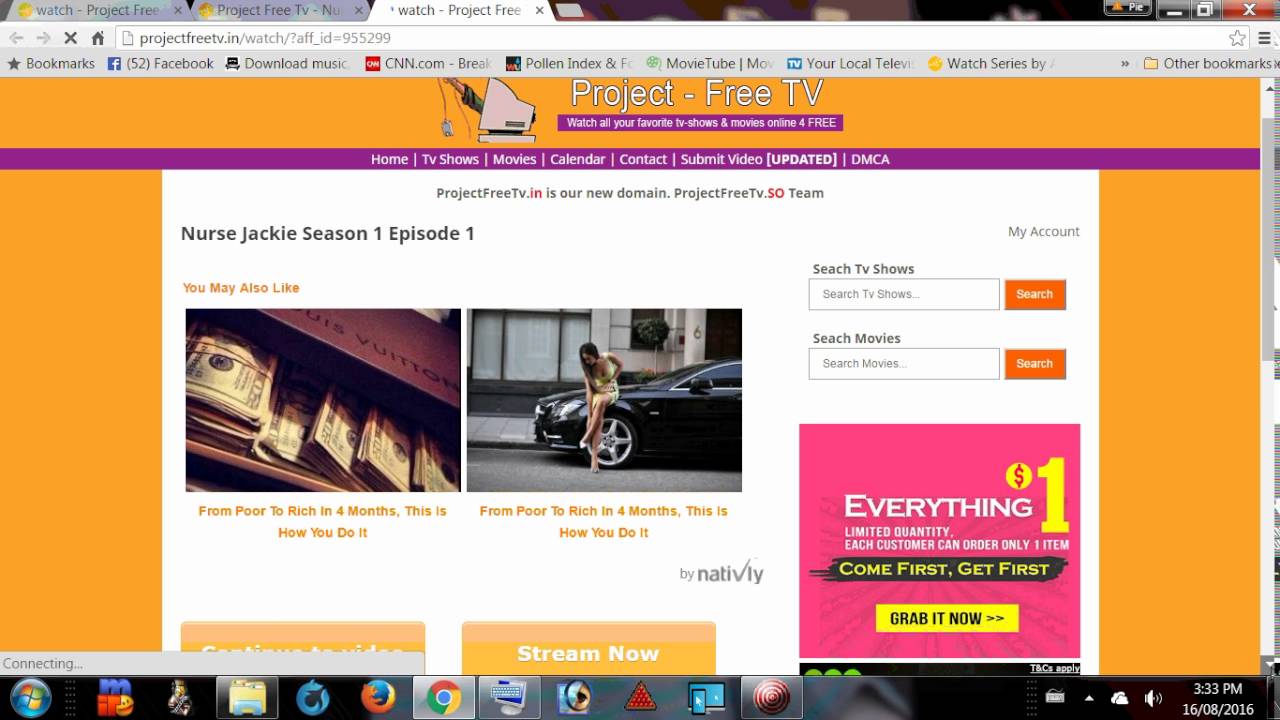A screenshot of a computer screen displays a fully opened web browser with three active tabs. The focused tab belongs to the website "Watch Project Free TV," with the URL reading "projectfreetv.in/watch/?AFF_ID=955-299." The webpage features a yellow background and showcases the Project Free TV logo prominently at the top. The logo depicts an old CRT monitor with an arm extending out, holding a computer mouse. Directly beneath the logo, in a purple rectangle with white text, the slogan reads: "Watch all your favorite TV shows and movies online for free," with "for free" written as "4FREE" in capital letters.